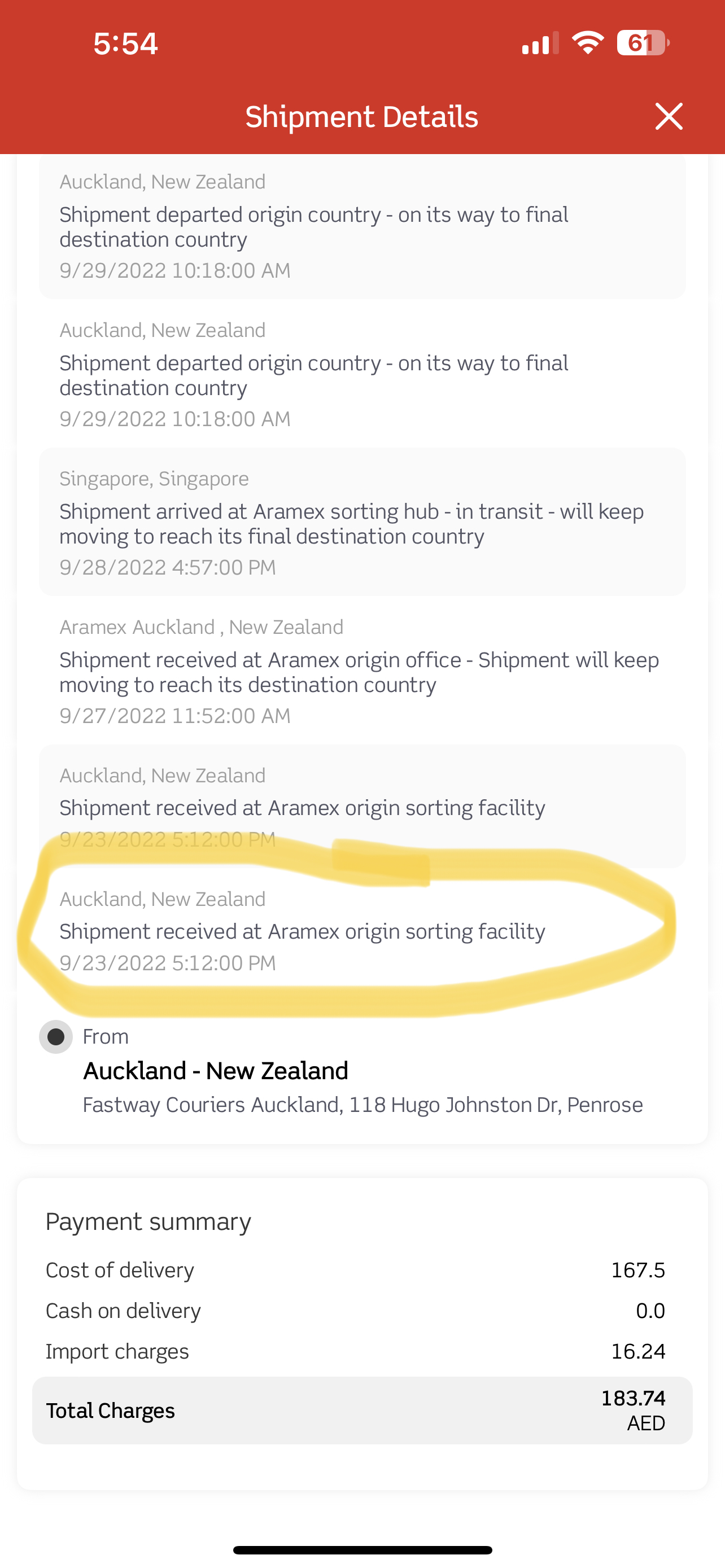A screenshot from a mobile email app displays a detailed shipment tracking update. At the top, the device clock shows 5:54, and the status bar on the right indicates Wi-Fi connection, signal strength, and a battery life at 61%. Below this bar, a red banner with white text reads “Read Shipment Details,” accompanied by a white 'X' on the right side.

The main content is set against a white background with text in gray and black. At the top, bold text indicates the shipment’s progress listed step by step:

1. **Auckland, New Zealand:** Shipment departed origin country, en route to final destination, **09-29-2022, 10:18 AM.**
2. **Auckland, New Zealand:** Shipment departed origin country on final leg, **09-29-2022, 10:18 AM.**
3. **Singapore, Singapore:** Shipment arrived at Aramex Sorting Hub, in transit to final destination, **09-28-2022, 4:57 PM.**
4. **Auckland, New Zealand (Aramex):** Shipment received at Aramex origin office, in transit to final destination, **09-27-2022, 11:52 AM.**
5. **Auckland, New Zealand:** Shipment received at Aramex Origin Sorting Facility.

A specific part of the text—“Auckland, New Zealand, shipment received at Aramex Origin Sorting Facility, 09-23-2022, 5:12 PM”—is highlighted in yellow, suggesting a noted detail.

Towards the bottom, the screen displays the sender’s information, encased in a circled checkbox: **“From: Auckland, New Zealand, Fastway Couriers, Auckland, 118 Hugo Johnson Drive, Penrose.”**

Following this, a section labeled “Payment Summary” outlines the costs associated with the delivery:
- Cost of delivery: **167.5 AED**
- Cash on delivery: **0.0 AED**
- Import charges: **16.24 AED**
- Total charges: **183.74 AED**

This comprehensive view provides clear insight into the shipment’s journey and associated costs.